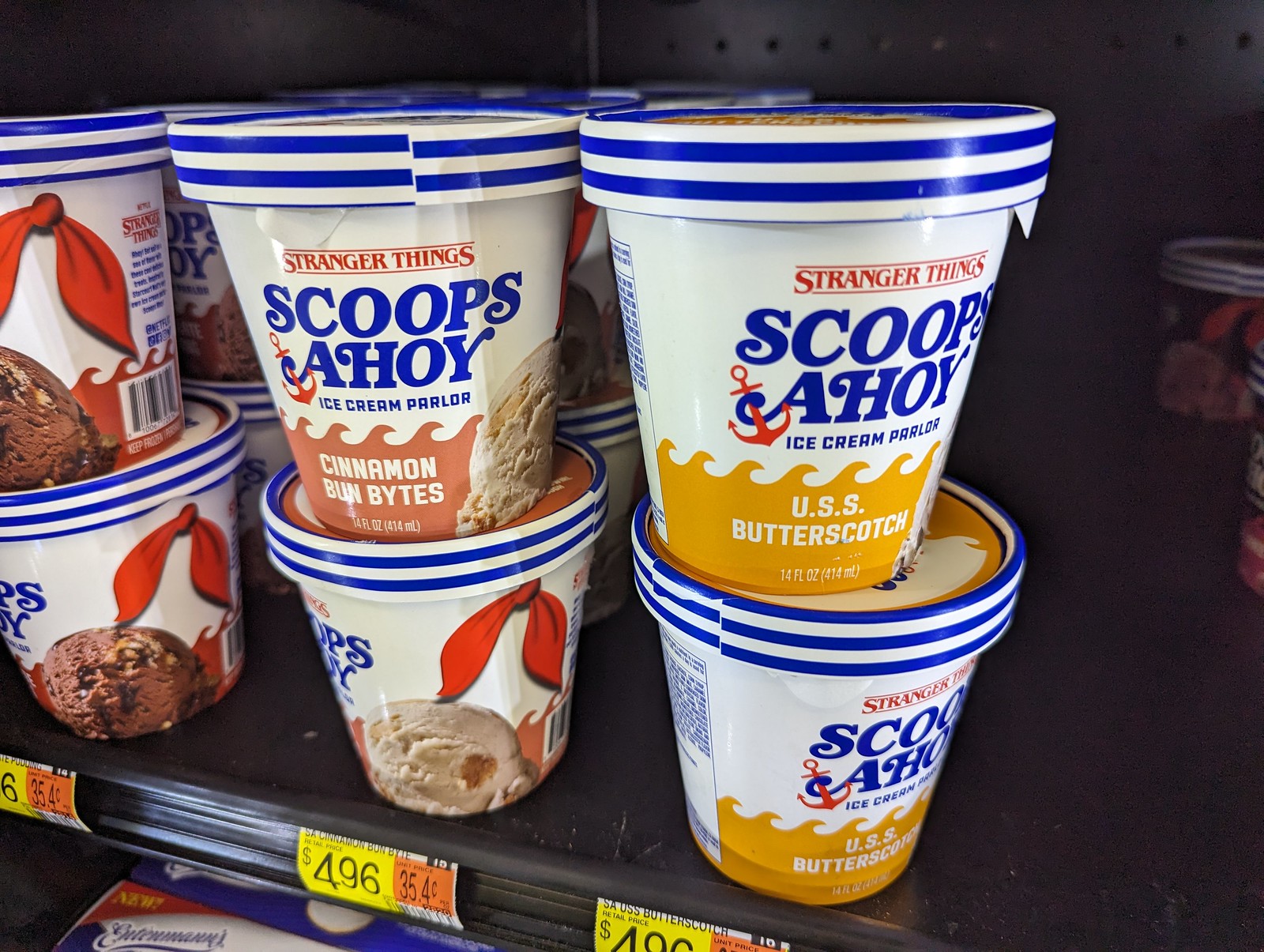The photograph captures a black supermarket shelf adorned with green and yellow price tags providing details such as cost per liter. Prominently displayed on the shelf are cartons of premium ice cream in the shape of circular containers, stacked in three columns with two containers in each column. These ice cream cartons bear the label "Stranger Things, Scoops Ahoy, Ice Cream Parlor" and include various flavors—on the left, a chocolate variety adorned with a red ribbon featuring crunchy pieces; in the center, 'Cinnamon Bun Bites' with a tan-colored ice cream mixed with cinnamon hues; and on the right, 'USS Butterscotch.' The price tag shows $4.96 with a unit price of 35.4 cents per ounce. Below this shelf lies another one holding a box of Entenmann's desserts in a cooler, signaled by a red 'New' sign with yellow font, situated against a predominantly blue and white container backdrop. The bottom left of the photograph reveals the shelf’s end, and towards the right, an empty section of the shelf is visible.